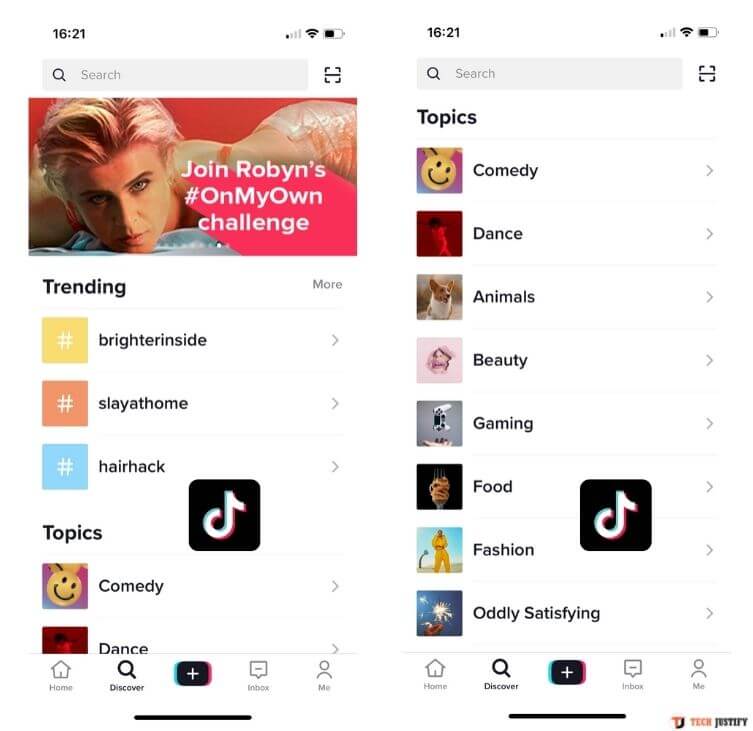The image depicts a screen from a social media or entertainment website, shown in a mobile interface layout. 

In the top left corner, the time is displayed in military format as 16:21. To the right, a signal bar shows one bar of strength, followed by a full Wi-Fi icon and a half-full battery icon.

Beneath this status bar is a rectangular search area with a magnifying glass icon on the left and the text "Search" next to it. To the right of the search bar is a small barcode camera icon, presumably for scanning QR codes.

Below the search bar is a heading that says, "Join Robin's #OnMyOwn Challenge," accompanied by an image of a male lying down and looking outside the picture frame.

Further down, a "Trending" section lists topics such as "Brighter Inside," "Slay," "A Thong Hair Hack," each with arrows pointing to the right, likely indicating ongoing trends or clickable links for more information. The familiar TikTok logo occupies the center of this section.

On the left side, there's a "Topics" category with "Comedy" listed first. The word "Dance" is cut off at the edge of the image, highlighting the user's interest or trending categories.

The right side shows another almost identical phone screen layout that extends the "Topics" category, listing "Comedy," "Dance," "Animals," "Beauty," "Gaming," "Food," "Fashion," and "Oddly Satisfying," each accompanied by relevant icons.

At the bottom of the screen, universal navigation icons for "Home," "Discover," "Inbox," and "Me" suggest standard features of the app, forming the basis for user interaction and exploration on the platform.